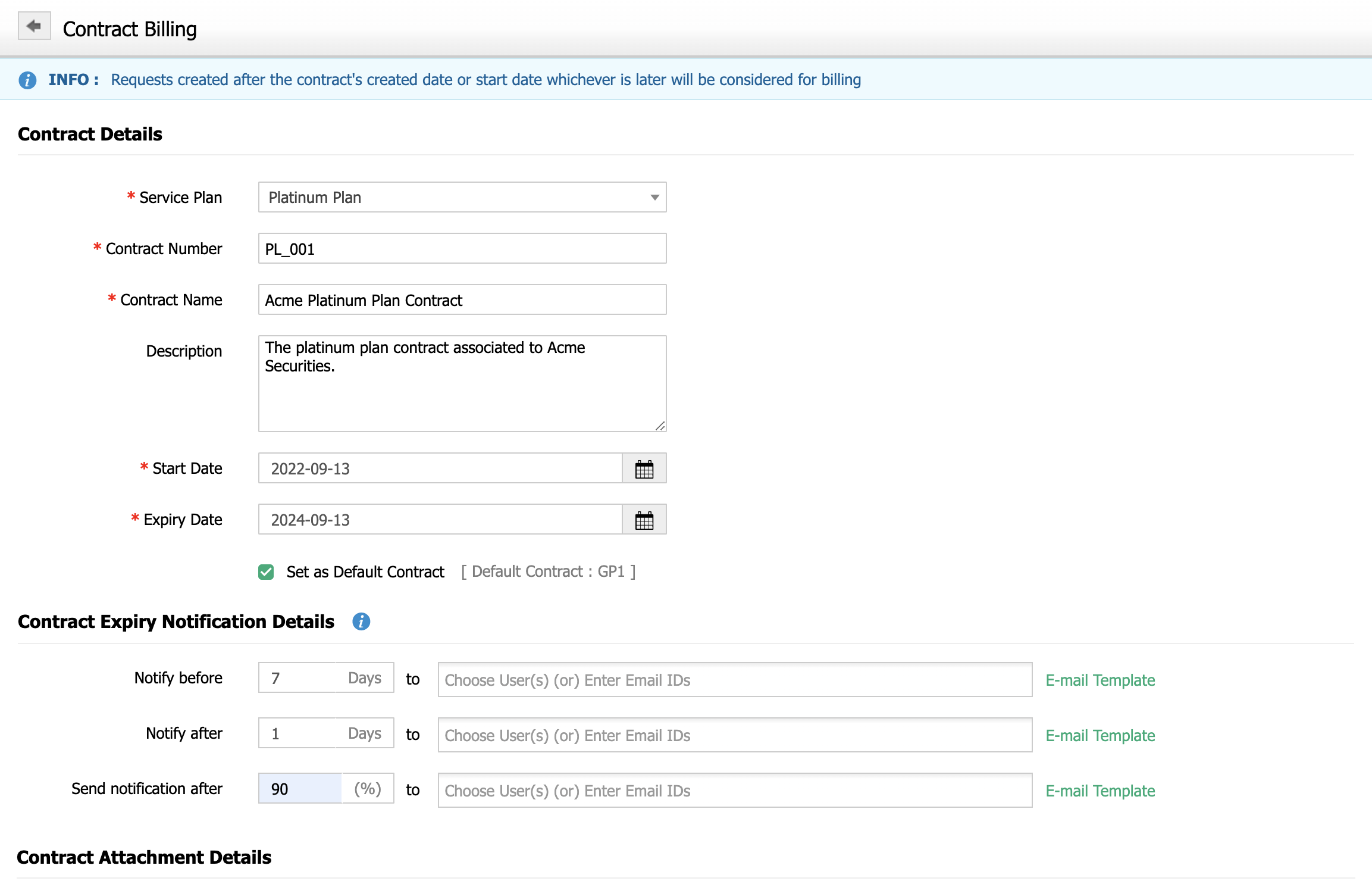**Detailed Caption:**

The image displays a section of a website dedicated to contract billing. At the top, an arrow is visible, allowing users to navigate back to the previous page. The page header indicates the category "Contract Billing". 

Beneath the header, there is a light blue notification bar containing the message: "Requests created after the contract's creation date or start date, whichever is later, will be considered for billing."

Below this message are the contract details, including:
- **Service Plan:** Platinum Plan
- **Contract Number:** PL_001
- **Contract Name:** ACME Platinum Plan Contract
- **Description:** This is the Platinum Plan contract associated with ACME Securities.
- **Start Date:** September 13, 2022
- **Expiration Date:** September 13, 2024 (indicating a two-year duration).

There is also a checkbox labeled "Default Contract," which is selected.

Following the contract information, there are fields for contract expiry notifications, including:
- Notify **before** 7 days to (email field for entry).
- Notify **after** 1 day to (email field for entry).
- Send notification **after 90%** completion to (user selection field).

Lastly, the section "Contract Attachment Details" seems to offer additional options for billing and communication regarding the contract. An information icon is available for users to click for more detailed explanations.